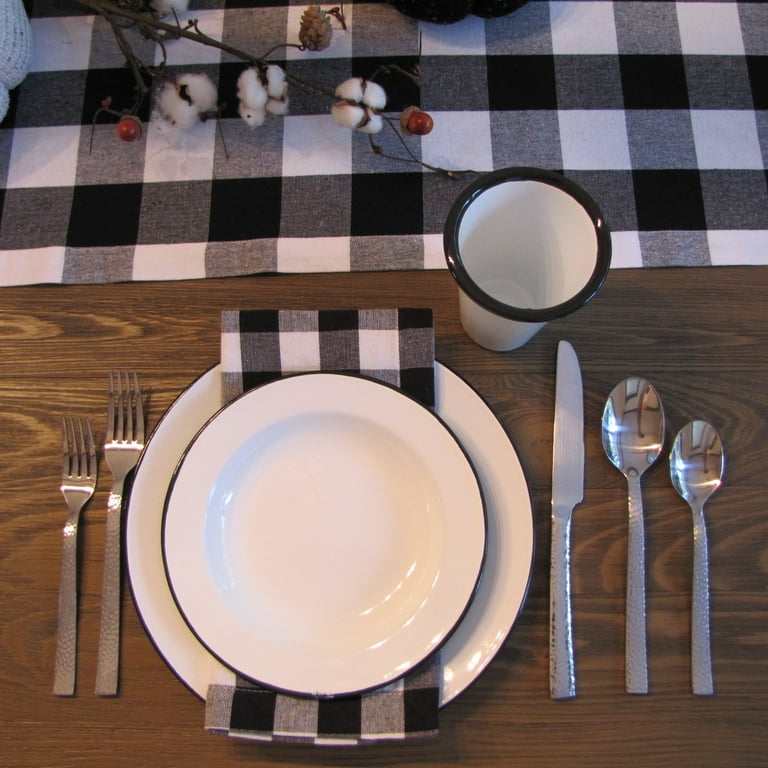This photograph captures a detailed place setting on a medium-colored wooden table. At the top of the image, a black-and-white checkered table runner extends horizontally, accompanied by a decorative black stem adorned with small cotton pieces and red-topped acorns. Below this, we see a white cup with a black rim situated in the upper right hand corner. 

Central to the composition is a layered arrangement of plates: a larger white plate with a black rim forms the base, topped by a slightly smaller white plate also rimmed in black, and finally, a shallow white bowl with a black rim resting on top. Between the plates, a neatly folded black-and-white checkered napkin mirrors the table runner above.

The cutlery is meticulously arranged: to the left of the plates, a larger fork and a smaller fork lie parallel, with the larger fork positioned closer to the plates. On the right, a butter knife is followed by a larger spoon and then a smaller spoon, all made of chrome.

This well-organized setting emphasizes a monochromatic theme while adding visual interest through its layered elements and the unique combination of rustic wooden texture and polished dinnerware.